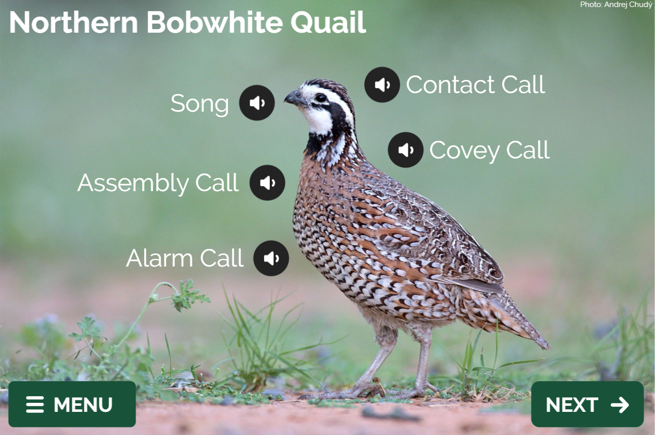The image depicts a detailed screenshot from an application or website, showcasing a northern bobwhite quail as the main focus. The bird, identified by its white font label at the top, exhibits a diverse coloration: a black and white head with additional black markings around the eye, a small black beak, and a mix of brown, light brown, white, and gray feathers across its body. The quail is standing on the ground amidst some grass and dirt, in a softly lit environment with diffuse light and no sharp shadows.

Surrounding the quail are several small black icons featuring white speaker symbols. These icons are labeled with different audio cues such as "Song," "Assembly Call," "Alarm Call," "Contact Call," and "Covey Call," suggesting that clicking each icon will play the respective sounds made by the bird.

In the interface, the bottom left corner features a green rectangle containing a white hamburger icon labeled "Menu," while the bottom right corner includes a similar green rectangle with the word "Next" in white, accompanied by a right-pointing arrow.